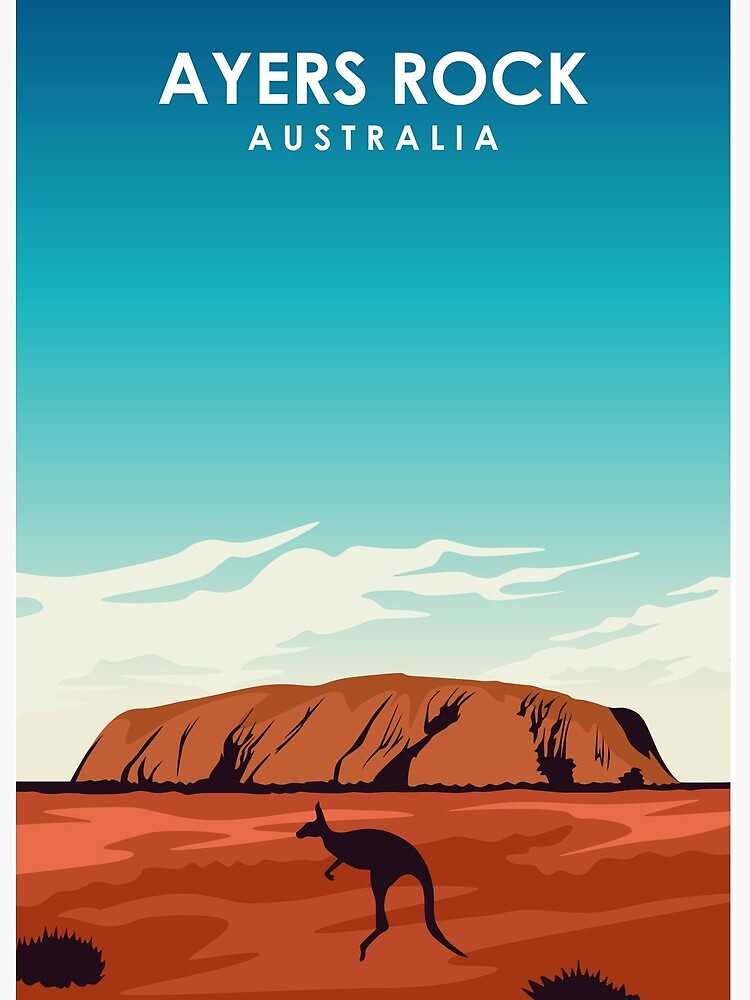This animated image appears to be a computer-generated art piece, potentially used as a cover for a book, brochure, or travel pamphlet about Australia. Prominently displayed at the top are the words "AYERS ROCK, AUSTRALIA" in bold, all-white capital letters. The background features a gradient blue sky, transitioning from a bright blue near the horizon to a darker blue at the top, adorned with a few scattered white clouds. Dominating the center of the image is a large brown rock formation, likely Ayers Rock, accented with black textured designs. The foreground consists of a reddish-brown desert landscape, where we see black silhouettes of plants and brush on either corner. The main focal point includes the black silhouette of a kangaroo in mid-leap, oriented towards the left side of the scene. Details such as the texture on the rock, the distinct layers of the sky, and the dynamic pose of the kangaroo add depth and interest to this visually striking depiction of Australia's iconic landscape.